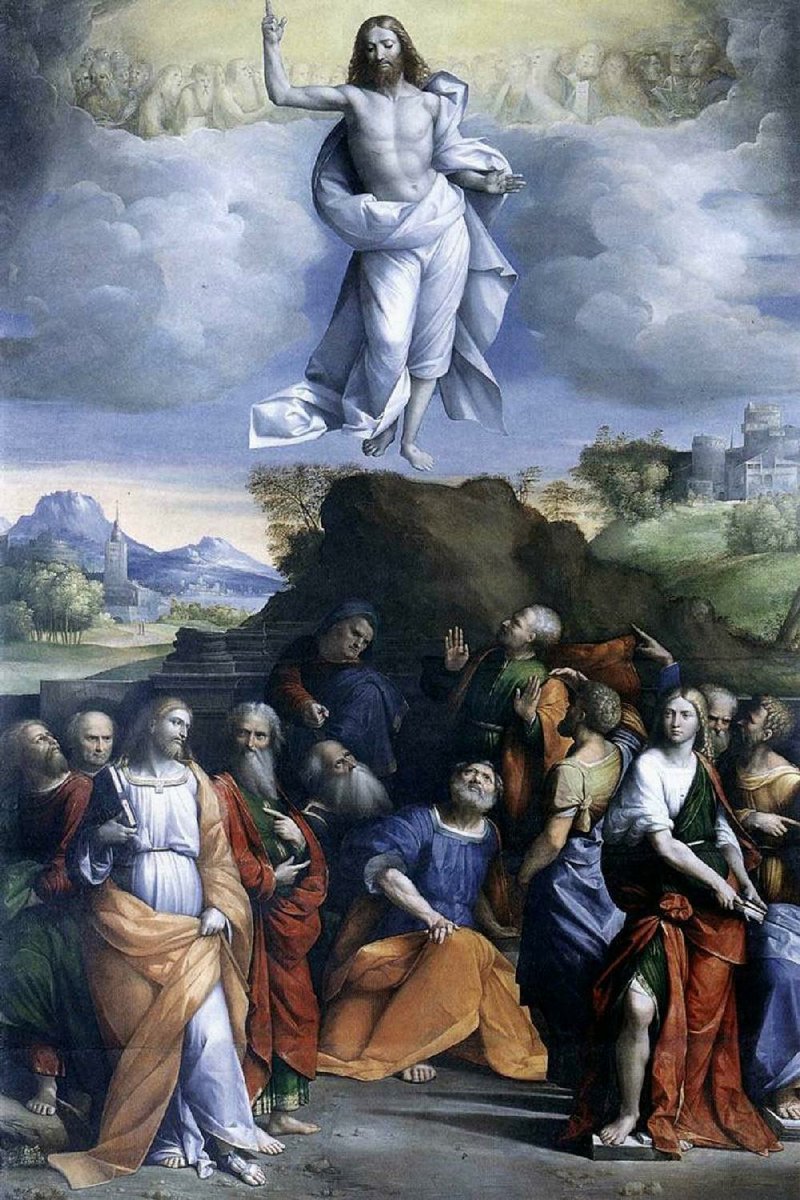The image depicts an artistic representation of the ascension of Jesus Christ, rendered in a style reminiscent of classical or medieval eras. Jesus, distinguished by his long brown hair, beard, and bare chest, is depicted floating in the sky, draped in a white robe that swirls around his waist and legs. His right arm is raised, elbow bent, with one finger pointing upward, and his eyes are closed in a serene expression. Surrounding him are ethereal, ghostly figures, perhaps representing ascended souls, partially obscured by white and yellowish clouds, suggesting a heavenly realm.

Below Jesus, a group of thirteen vividly drawn figures, likely the Apostles, are gathered in various postures of awe and conversation. They are attired in colorful, flowing garments—robes in red, blue, orange, and white—emphasizing the rich textile traditions. One central figure in a blue smock with an orange garment draped over looks up intently, while others exhibit a mix of reactions—ranging from looking upward, talking amongst themselves, to looking ahead or down.

The background of the image reveals a dynamic landscape with a rocky hill, verdant fields, and distant trees. On the left, stone buildings and a church steeple rise against a backdrop of mountains and an orangish sky, indicative of dawn or dusk. The realistic countryside contrasts with the ethereal upper scene, grounding the divine occurrence in a familiar earthly setting. Overall, the painting encapsulates the mystique and reverence associated with the ascension of Christ, weaving together elements of the divine and the terrestrial in a single, cohesive tableau.